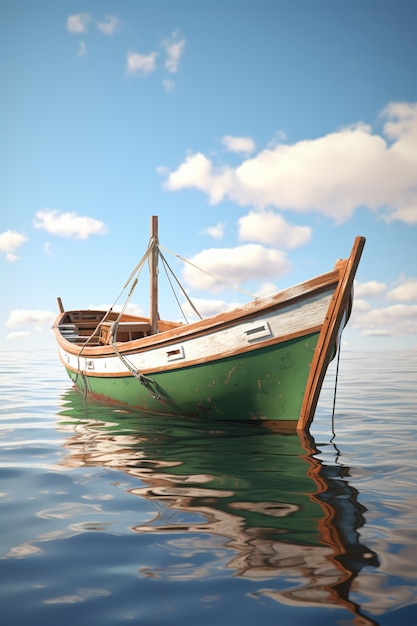This vertical rectangular photograph captures an up-close view of a very old, green-painted wooden sailboat anchored in calm, dark blue ocean waters, gently rippled enough to create a reflective surface. The boat’s structure prominently features a brown wooden mast in its center, devoid of sails, rising from a higher central brown wooden box. The boat's hull is green with a contrasting white strip running across the top, and scupper drains marking the hull. The side and front views reveal the wooden keel and several ropes, including an anchor line descending from the prow into the water. Above, the daytime sky is a vibrant blue adorned with cottony white clouds, adding a tranquil ambiance to the scene.